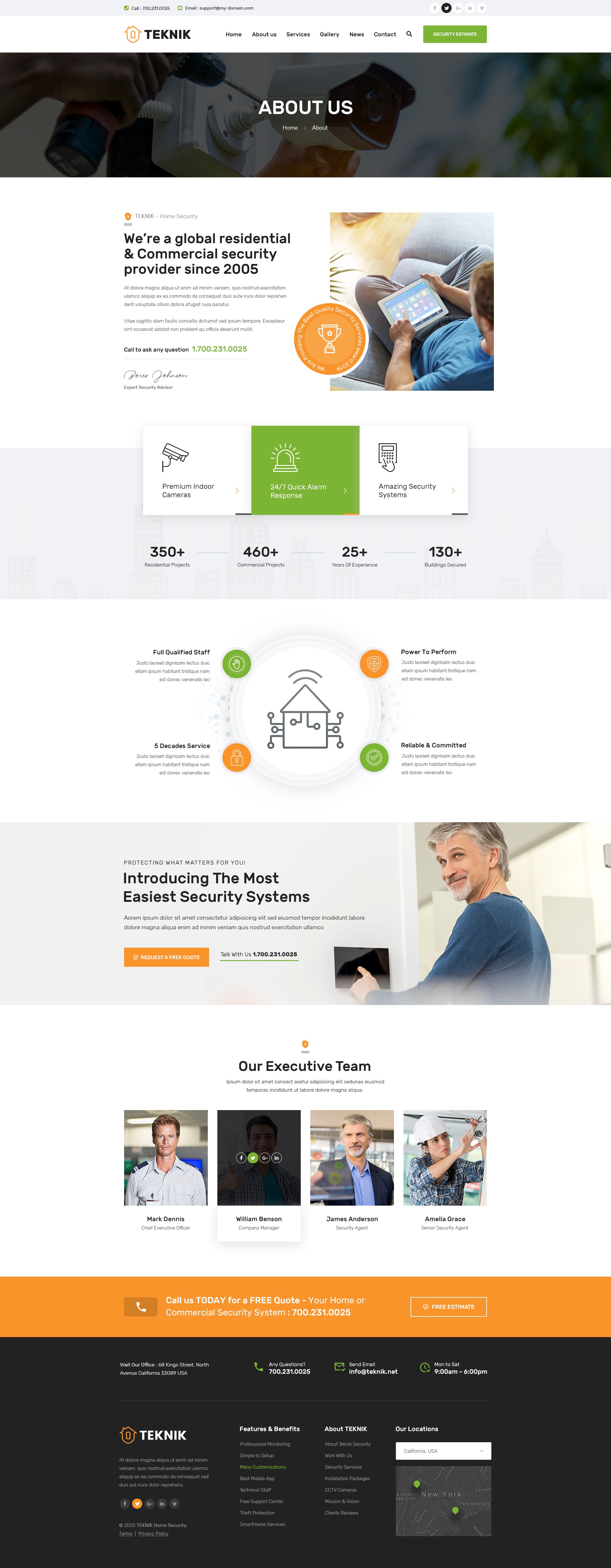This is a detailed and comprehensive description of a website template for a security service provider named "Technik." At the very top, you will find the logo featuring the name "Technik" (stylized as T-E-K-N-I-K) with an orange house outline and a badge icon to the left. The header includes six menu options, which are not clearly legible, and social media icons. To the right, there is a prominent green button with an unreadable label.

Just below the header, the "About Us" section confirms the company's global presence in residential and commercial security since 2005. This section features an image of an individual installing security cameras on a wall, though the picture is darkened by a transparent black overlay. A statement sits beneath the image, declaring their global provider status.

Next, the website showcases an overhead shot of a man resting on a couch and using an iPad to control some kind of interface. Adjacent to this visual, icons of a camera, an alarm, and a keypad are displayed, accompanied by various statistical figures: over 350 installations, over 460 of some unspecified metric, and two additional figures related to their services.

The color scheme prominently features green and orange hues. In the middle of the page, a green panel highlights alarm systems. Nearby, an orange circle with a trophy signifies some form of accolade or recognition. 

The subsequent section uses an illustration of a house to demonstrate interconnected security features, with four key points accompanied by icons in green and orange.

Further down, an image of a man likely in his 40s introduces the user-friendly nature of their security systems. Following this, the executive team is presented with four thumbnail images, with some members shown working in the field.

The footer of the website is extensive, containing site navigation links, social media icons, a map, and contact information, although the text is small and hard to read.

Overall, the website template is visually rich, but it contains an overwhelming amount of information that requires scrolling to fully view.